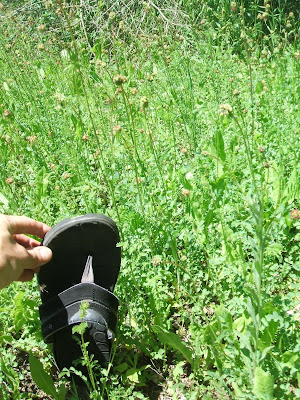The image captures a dense field of tall, yet-to-bloom flowers, their maturity evident despite the unopened buds. Prominently featured in the foreground, a white individual’s partially visible left hand holds a rugged black flip-flop with thick soles and substantial top support. The person's hand, visible from just above the thumb, highlights the comparison of the flip-flop’s height against the flowers, revealing that the blossoms reach about half the length of the footwear. The field, almost entirely blanketed by the flowers, shows a variety of green leaves sprouting from the base of the plants and extending towards the ground, creating a lush and vibrant setting. The image is saturated with greenery, filling around 80% of the frame.